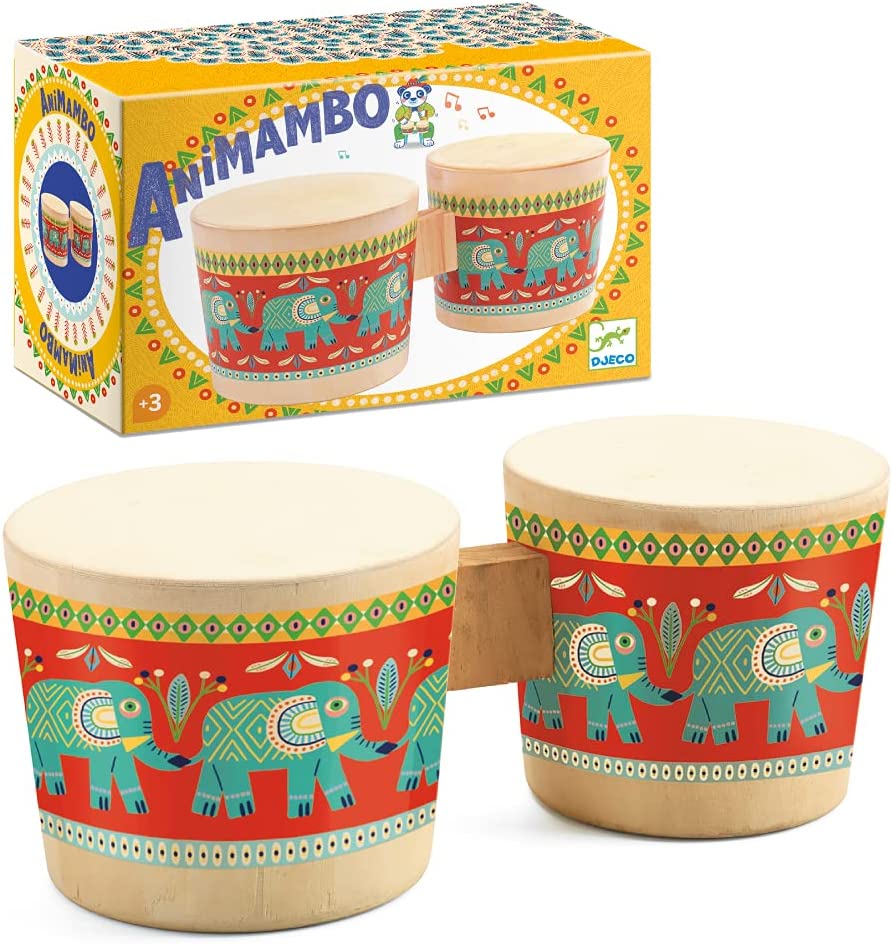The image showcases a retail display of a children's toy drum set called Animambo, suitable for a toy store or for sale on a retail website. At the top left of the image, there is a vibrant yellow box adorned with intricate blue designs. The box prominently features the name "Animambo" in bold blue letters. Accompanying the text is a playful illustration of a bear playing the drum, wearing a red hat and blue jeans. Below "Animambo," the brand name "DJECO" with a lizard logo appears on the bottom left of the box.

In front of the box, the drum set is displayed, consisting of two small bongos connected by a wooden piece. The drum skins are white, decorated with red circular patterns and green diamond graphics. Each drum prominently features artistic depictions of teal-colored elephants marching in a line, exuding an artisan or native art style. The detailed illustrations include three elephants on one drum and a couple more on the other, creating a vibrant, playful design that stands out against the red backdrop. Additionally, the drums have small dot patterns encircling the base, enhancing their engaging, whimsical appearance.